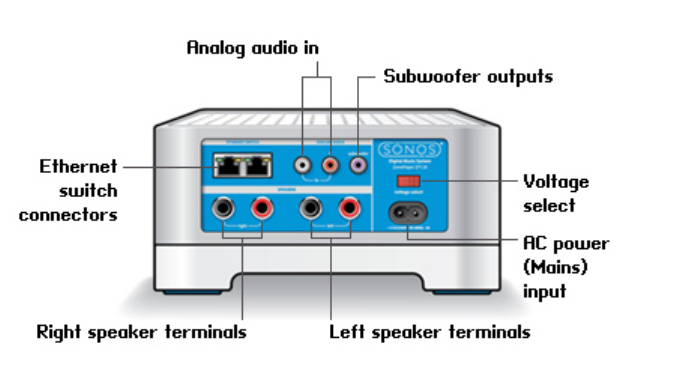The image depicts a detailed, digitally illustrated diagram of the back panel of a stereo amplifier. The panel, colored in blue and white, features numerous inputs and outputs arranged in a specific pattern. Starting from the top left, the panel includes two black slots marked as Ethernet switch connectors, followed by three circular inputs colored white for analog audio in (left), red for analog audio in (right), and purple for the subwoofer output. Towards the middle, there is a prominent red button labeled as the voltage select switch. Below this button, there is an AC power mains input connector. At the bottom left of the panel, two sets of black and red input terminals are designated for the right speaker (left pair) and the left speaker (right pair) respectively. The diagram also features labels in bold black font with arrows pointing accurately to each connector and terminal. Overall, this detailed description emphasizes the structured layout and specific functions of each component on the amplifier's back panel.